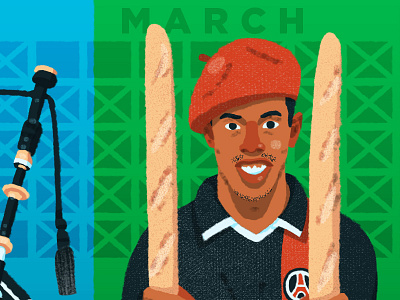This vibrant illustration prominently features the word "March" at the top in bold lettering. Below it, a man wearing a beret and a polo shirt with a decorative stripe running down the right side from his shoulder to the bottom of the frame is depicted. The polo shirt also features an emblem of the Eiffel Tower. The man holds two baguettes, positioned upright on either side of his face, with only the tops of his hands visible. He is shown from the chest up against a green background. To his right, there is a separate blue block showcasing what appears to be the top of bagpipes, adding an intriguing juxtaposition to the scene.